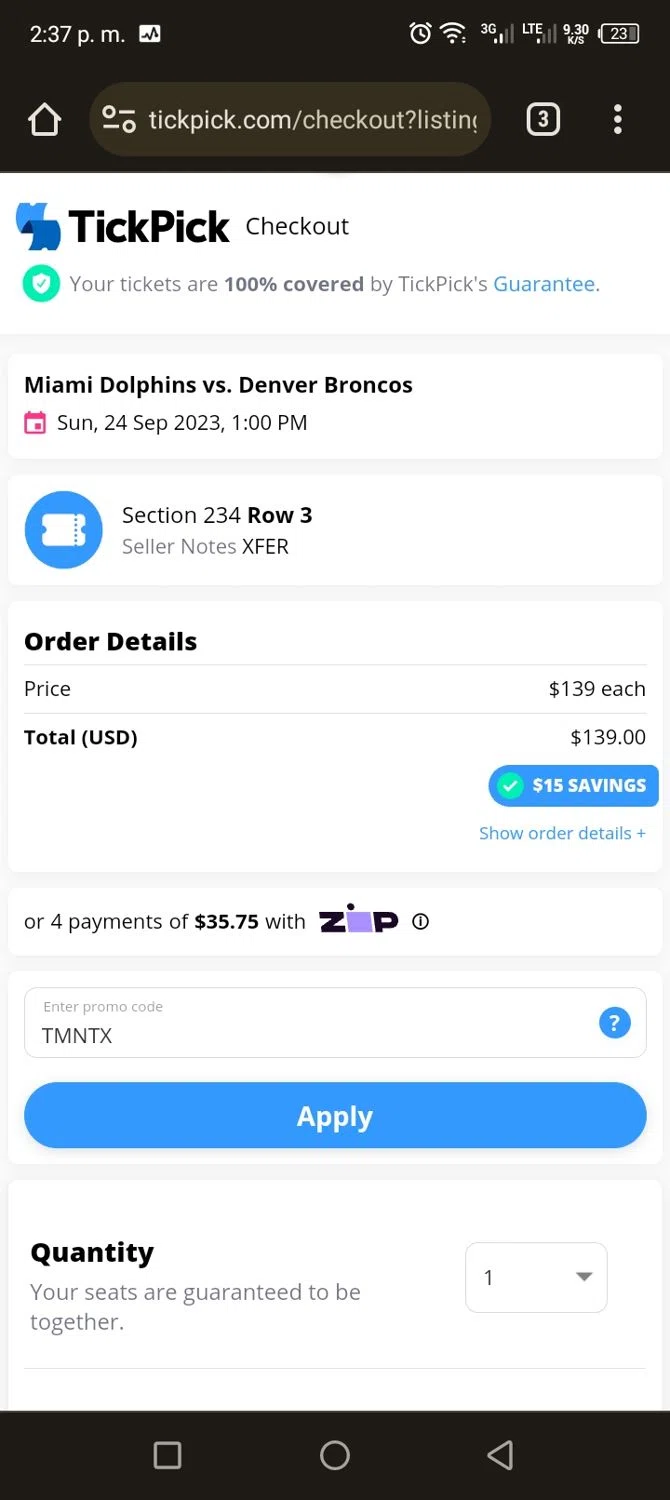**Image Caption:**

This vertical screenshot appears to be taken from a smartphone displaying a Ticket Selection or Checkout page for an event. At the top of the image, there is a black rectangle with the current time, "2:37 p.m." displayed in white text on the upper left side. On the upper right, icons indicating the clock, Wi-Fi strength, LTE connection, and battery life at 23% are present. 

Below the black rectangle, on the upper left, there's an icon resembling a house next to a gray bar where the web address "TickPick.com/checkout?listing" partially displays, followed by a small white square with the number "3" in it. On the upper right side, three vertical dots symbolize more options.

Moving further down, the title "TickPick Checkout" is visible, accompanied by a green icon with a white check mark, indicating the guarantee that the tickets are 100% covered by TickPick. The event details are Miami Dolphins versus the Denver Broncos, scheduled for Sunday, September 24, 2023, at 1:00 p.m., in Section 234, Row 3.

Additional information includes:
- Seller notes indicating the tickets are to be transferred.
- The order details mention the price per ticket at $139, reflecting a $15 savings.
- Options to view order details or opt for installment payments of $35.75 each, represented by a 'Z' in a purple square followed by 'P'.
- A field to enter a promotion code labeled "T-M-N-T-X" with an apply button.
- Quantity selector ensuring seats are guaranteed together, currently showing "1".

At the bottom of the screenshot, a large black box is visibly prominent.